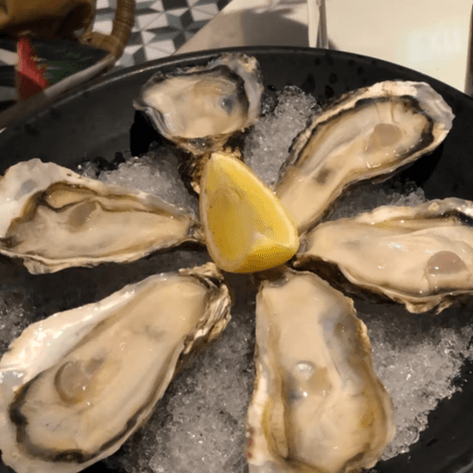This square-shaped image captures a top-view of a neatly arranged culinary presentation. At the center, a black frying pan holds six oysters on the half shell, symmetrically positioned to radiate outwards like flower petals, anchored by a bright yellow lemon wedge at the core. Each oyster, resting on a bed of crushed ice, displays a beige to grayish body framed by a white and brown-rimmed shell. The crushed ice nestles between the shells, enhancing the dish’s freshness. The pan's glossy black surface contrasts sharply with the pale oyster shells and ice. Surrounding the focal point, the background reveals a tiled floor featuring a distinctive star pattern within a white square, rendered in charcoal and black hues. The upper right corner includes a partial view of a wall, adding depth to the setting, while faint outlines in the backdrop suggest the presence of chairs, subtly framing the well-composed plate of seafood.